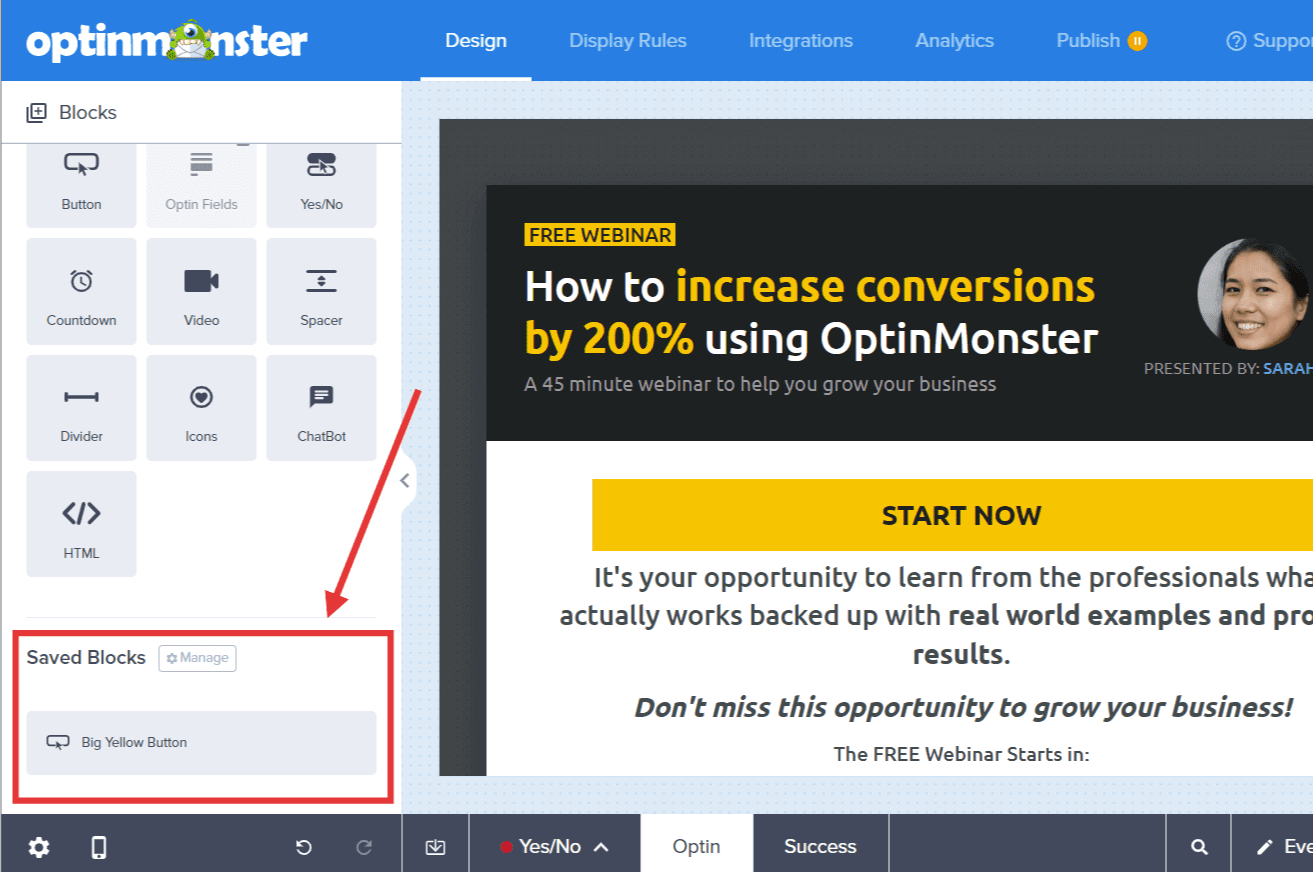This screenshot captures a web page belonging to a service or product called OptinMonster, as identified by the company logo located in the top left-hand corner. The logo features the word "OptinMonster" in a white-colored font accompanied by an image of a one-eyed green monster. 

At the top of the page, there are multiple navigation links. From left to right, they are labeled as follows: Design, Display Rules, Integrations, Analytics, Publish, and Support. These buttons provide access to various functionalities within the OptinMonster platform.

In the bottom left-hand corner, there is a section outlined with a red rectangle that highlights a feature labeled "Save Blocks." Next to this, a smaller button labeled "Manage" appears, also outlined with a red rectangle.

Dominating the upper right portion of the page is a prominent caption that reads: "Free Webinar: How to Increase Conversions by 200% Using OptinMonster." This is likely an announcement or advertisement for an upcoming webinar hosted by the company.